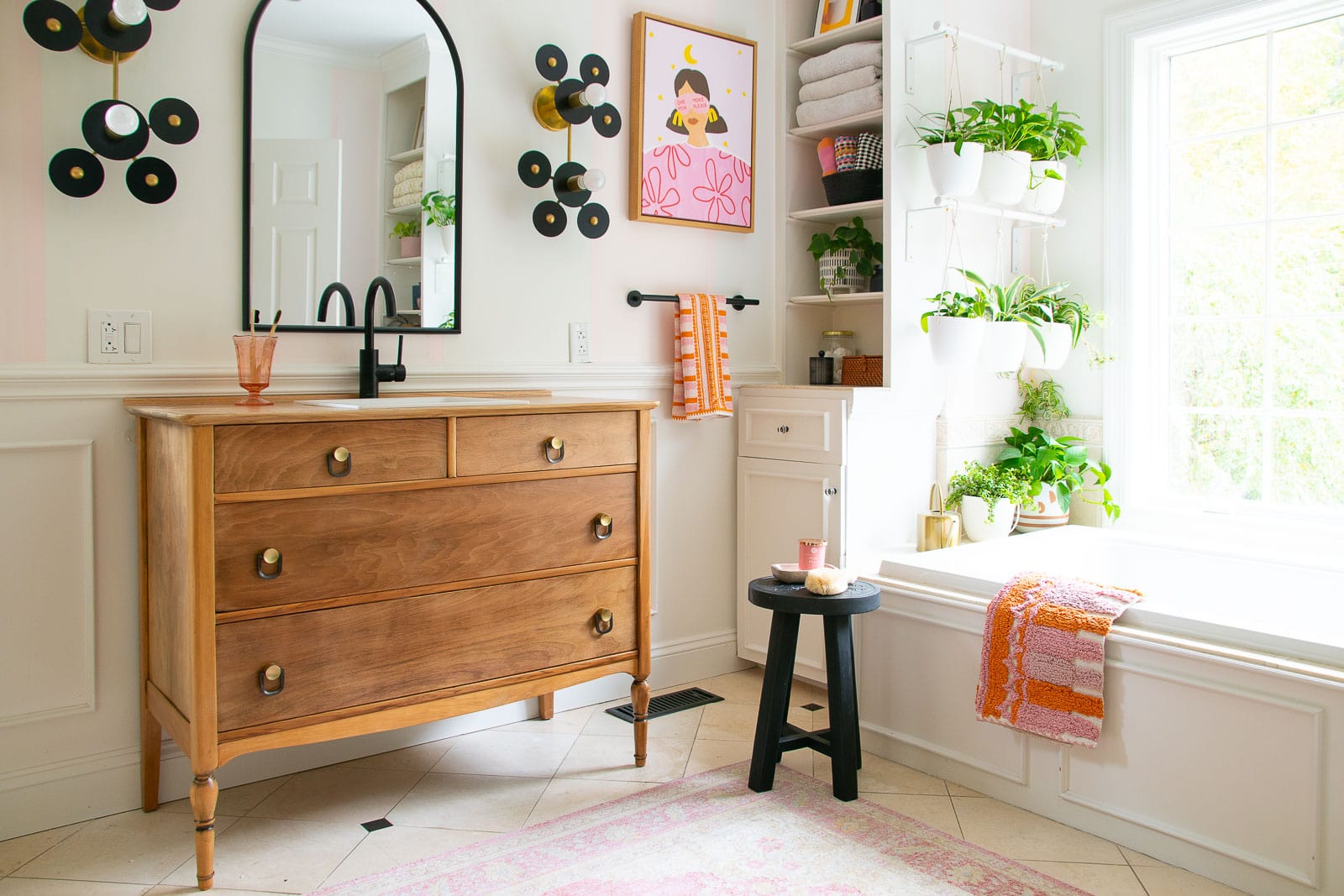The image depicts a stylish bathroom featuring a large bathtub positioned under a grid-patterned, white-framed window that reveals a view of trees outside. The bathtub is adorned with a multi-colored towel in shades of orange, pink, and white, draped casually over its edge. Surrounding the tub are various white pots containing green plants, some with gold accents, arranged on shelves and hanging, adding a touch of nature to the space. 

Adjacent to the bathtub, there's a simple black stool supporting a yellow sponge along with a candle and soap. The bathroom also includes a wooden dresser integrated with a black faucet and sink, accompanied by a black-framed mirror. Soft, white towels are neatly organized on the shelves above the white cabinets, and there are additional details like cotton balls and another candle. The floor is tiled, and a pink rug adds a splash of color, tying together this serene and inviting bathroom.